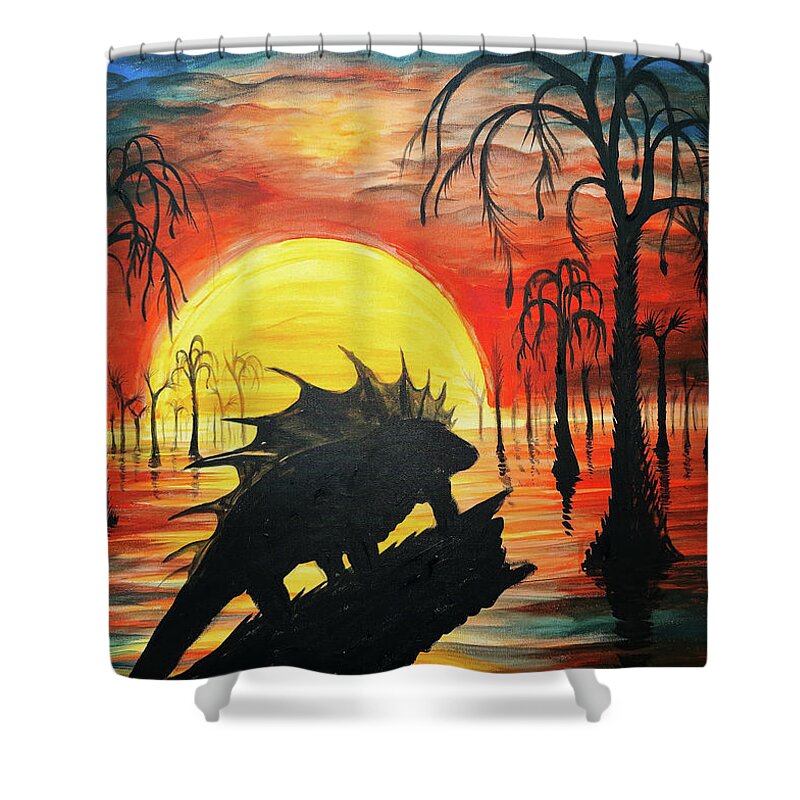The image is an artistic, square-shaped painting presented as a shower curtain hanging from black hooks on a white curtain rod, framed by gray borders at the top and bottom. The painting depicts an eerie, nighttime scene with a large, yellow sun or half-moon set against a vivid red sky that transitions to blue at the top. A dark, silhouetted iguana-like creature with spines along its back stands on a broken, black log amidst a body of water reflecting the vibrant sky. The water is interspersed with palm-like trees, appearing as black shadows. A mystical, eerie atmosphere permeates the scene, enhanced by the stark contrast between the bright sky and the dark silhouettes of the flora and fauna.